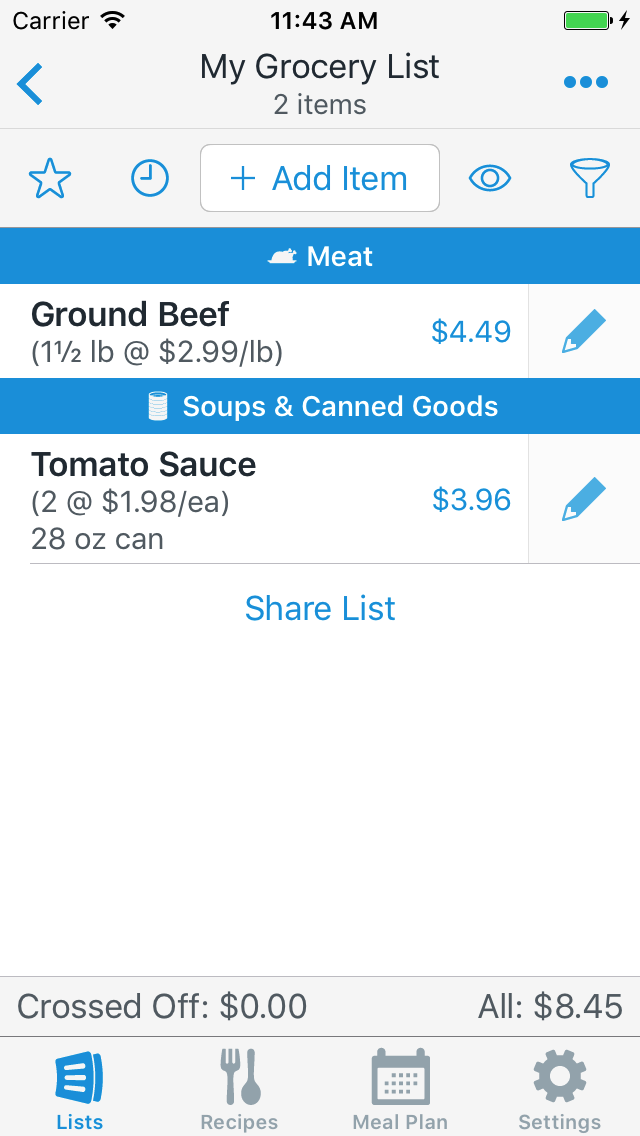The image is a screenshot from a smartphone, displaying the "My Grocery List" app interface. The phone's status bar at the top left reveals a full Wi-Fi signal and indicates the current time as 11:43 a.m., with the battery icon showing it is fully charged and plugged in.

The app interface is structured with a neat and organized list of grocery items. At the top, there's a function to star or favorite an item, and a white rectangular box with blue text that prompts users to "Add Item."

The first item on the list is categorized under a blue banner labeled "Meat," with "Ground Beef" listed in bold underneath. The details specify "1.5 pounds at $2.99 per pound," and next to this, in blue text, the total price of $4.49 is displayed. Adjacent to the item is a blue pencil icon, presumably for editing.

The second item falls under another blue banner labeled "Soups and Canned Goods." Here, "Tomato Sauce" is bolded, with the note "28-ounce cans at $1.98 each." The price of two cans is calculated and shown in blue as $3.96. Like the first item, a blue pencil icon is situated beside the tomato sauce for editing purposes.

Beneath the listed items, a button labeled "Share List" is visible. At the bottom of the screen, a gray banner shows "Crossed off $0," likely indicating items that have been marked as purchased. The total cost of the listed items is displayed as "$8.45" in blue.

Four navigation options are located at the bottom of the app: "List," which is highlighted in blue to indicate the current view, and "Recipes," "Meal Plan," and "Settings," all of which are in gray, suggesting they are inactive at the moment.